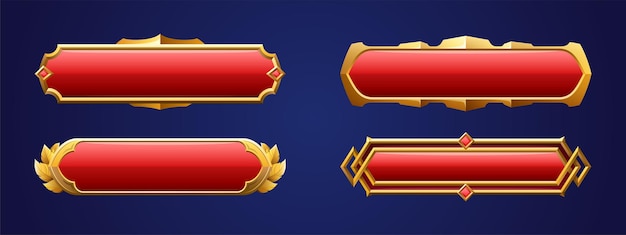This illustrated image features a dark royal blue background with a gradient that transitions from darker on the left and right sides to brighter in the center. Prominently displayed are four rectangular symbols, each characterized by a red gradient center and adorned with a metallic gold outline. Despite their shared red and gold color scheme, each symbol has a unique border design that sets it apart. The top left symbol's border is thinner compared to the others, thickening toward the top center and bottom center. The top right symbol features an art deco style. The bottom left symbol has a border concentrated on the left and right edges, with thin lines on the top and bottom. The bottom right symbol showcases an intricate art deco design, possibly with intertwining thin lines and diamond shapes. These symbols, reminiscent of ornate labels or nameplates, could potentially serve as decorative elements or buttons in a web design.